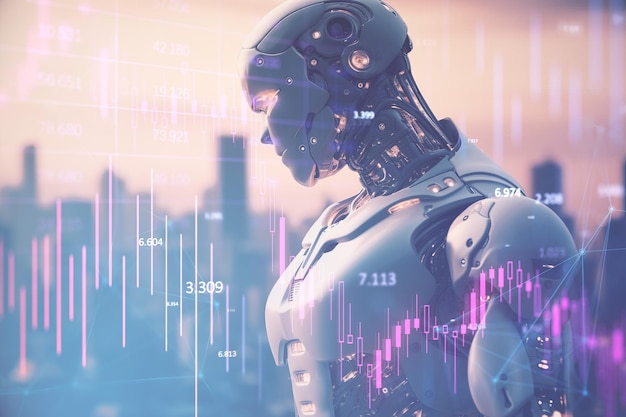The image depicts a detailed, computer-generated scene likely from a video game, featuring an android or cyborg that stands with its head lowered. The cyborg, feminine in appearance with visible breasts, appears to be constructed from both metal and plastic materials, and has a face shield that integrates seamlessly with its robotic visage. It resembles a less intimidating version of the Terminator robot, notable for its human-like features and metal composition. Blue digital numbers are displayed prominently on its body: 3.999 on its neck, 7.133 on its chest, 3.309 in front of its chest, and 6.974 on its shoulder, enhancing the high-tech feeling of the scene. Additional graphical elements include a purple bar graph under one shoulder and various vertical lines and numbers scattered across the screen, contributing to a computer display aesthetic. The backdrop is a cyberpunk cityscape with towering skyscrapers outlined in pink and white lines, set against a pink and black sky, augmenting the futuristic atmosphere of the image.